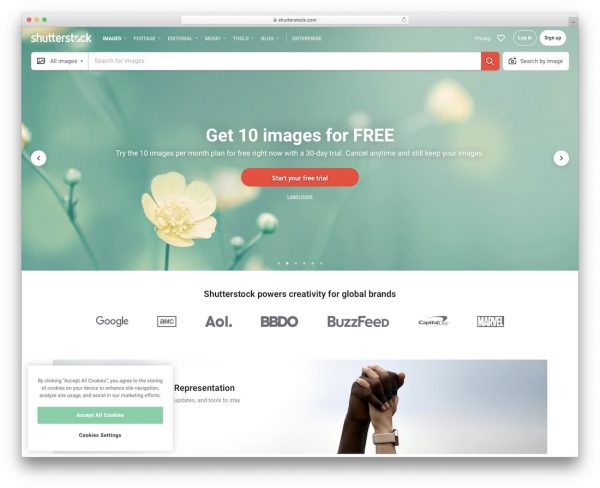The screenshot depicts a computer screen displaying the Shutterstock website. The traditional red, yellow, and green buttons for closing, minimizing, and maximizing the window are visible at the top left corner. The URL bar indicates the website address as Shutterstockshops.com. The centerpiece of the webpage is a slightly blurry image featuring a vibrant green background of vegetation with a flower in the foreground. At the very top of the page, the Shutterstock logo is prominently displayed, accompanied by various options including 'Share'.

To the far right, there are buttons to 'Like' content, alongside options to either 'Log In' or 'Sign Up' for users who don't have an account. Central to the page is a bold white text stating, "Get images for free," with further details listed below. A conspicuous red button invites users to "Start your free trial". An informative section beneath this button declares, “Shutterstock powers creativity for global brands like Google, AOL, BBDO, BuzzFeed, and others," emphasizing the platform's extensive influence. Completing the visual, an evocative image of two hands clasped together symbolizes unity and collaboration.